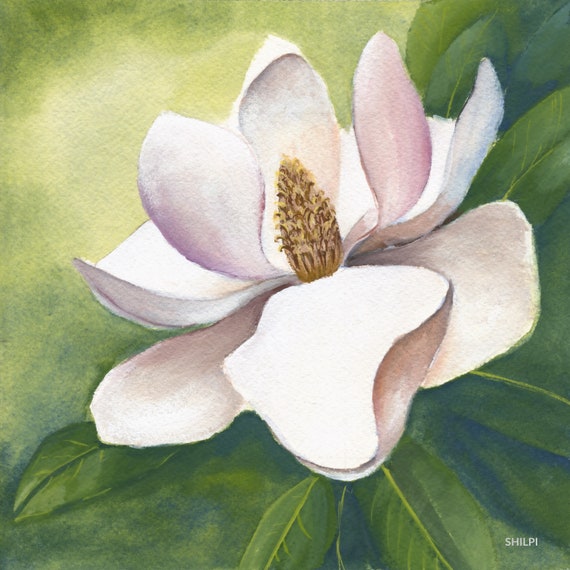This detailed painting captures a stunning white and pink flower, prominently centered and illuminated in a tropical outdoor setting. The flower features an almond-shaped core in shades of yellow and brown, surrounded by an array of teardrop and rounded-shaped petals, with some appearing folded back or concave. The texture and varying hues of the white petals, tinged with light pink, are meticulously highlighted. Encircling the flower are green leaves with visible veins and elliptical shapes, providing a textured contrast to the delicate petals. The background gently transitions from light yellow to white and green, emphasizing the flower's central position. At the very bottom right corner of the image, the artist’s signature, "SHIPI," is engraved in white uppercase letters, adding a final touch to this elegant artwork.